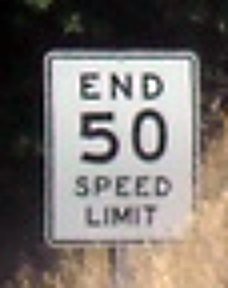The image depicts an extremely out-of-focus traffic sign situated against a predominantly black background with a patch of dry grass in the lower right corner. The large, white sign with a black border and background prominently displays the text "END 50 SPEED LIMIT." The word "END" is written in black text at the top, followed by a large number "50" in the center, and "SPEED LIMIT" stacked vertically beneath it. The visual clarity is compromised by noticeable artifacts surrounding the letters, accentuating the lack of focus and adding a layer of distortion to the overall scene.